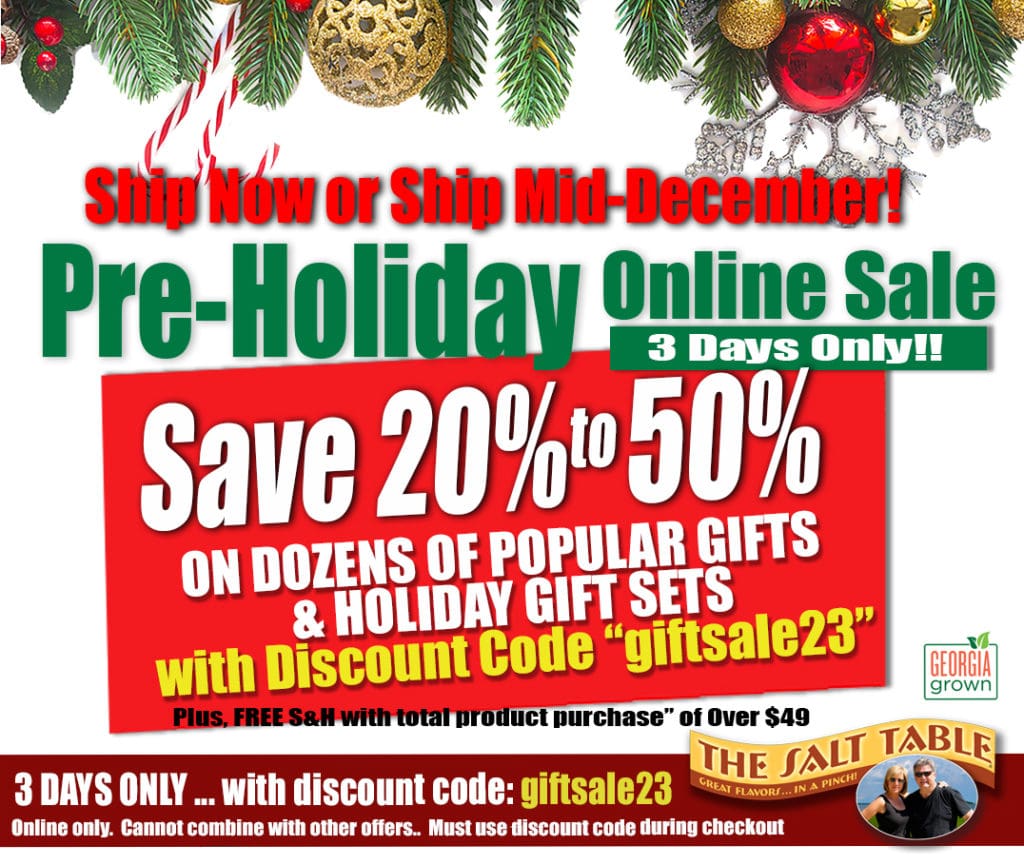This image features an advertisement with a festive, holiday-themed design. At the top, pine branches reminiscent of Christmas décor frame the text. Just beneath these branches, bold lettering instructs, "Ship now or ship mid-December." Following this, a prominent announcement declares a "Pre-Holiday Online Sale, Three Days Only." The main body of the ad emphasizes a significant offer: "Save 20% to 50% on dozens of popular gifts and holiday gift sets."

In the bottom right-hand corner, there's a small, wavy banner with text that reads "The Salt Table." This banner is notably smaller compared to the rest of the elements on the advertisement. Beside this text is a circular logo featuring two figures, a man and a woman, which suggests they are the owners or representatives of The Salt Table company. Above the banner, a tagline proudly states, "Great Flavors in a Pinch," reinforcing the brand's emphasis on quality and convenience. The overall design and color scheme evoke a warm, festive atmosphere, perfect for the holiday season promotions.